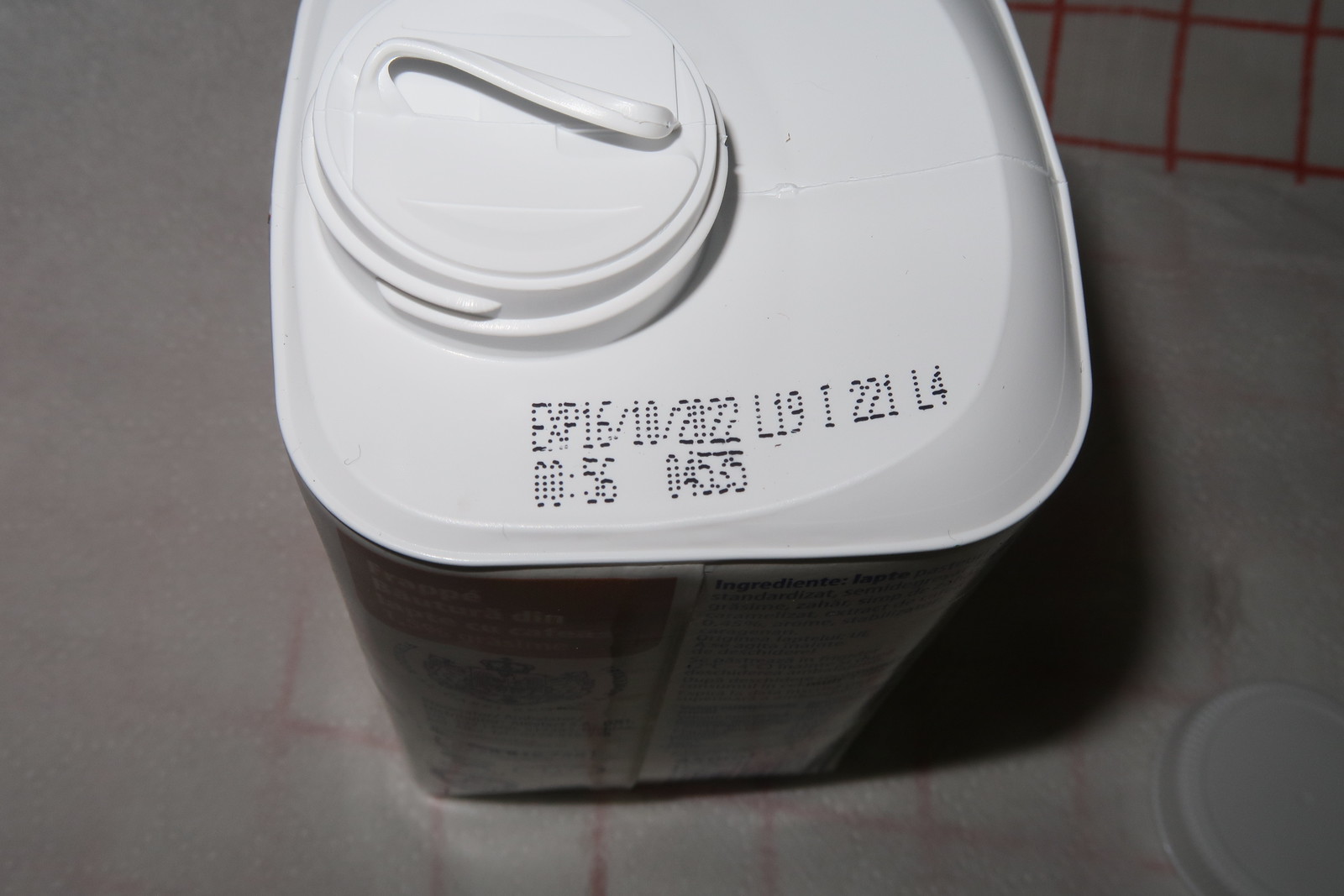The image shows a square white lid of a Tupperware-type container, viewed from above. The lid features a large hole on the left side, which is covered by what appears to be a screw-on cap. Stamped details across the top of the lid include the expiration date "16-10-2022," and a series of codes: "L19I221L4," "000056," and "04535." The container beneath the lid seems to be clear, revealing its contents—an object that appears to be a dark-colored mat possibly used for cooking, encased in plastic. A white lid is also visible on the right, edged in red with white sections inside the borders, which is a recognizable pattern often seen in cooking mats.